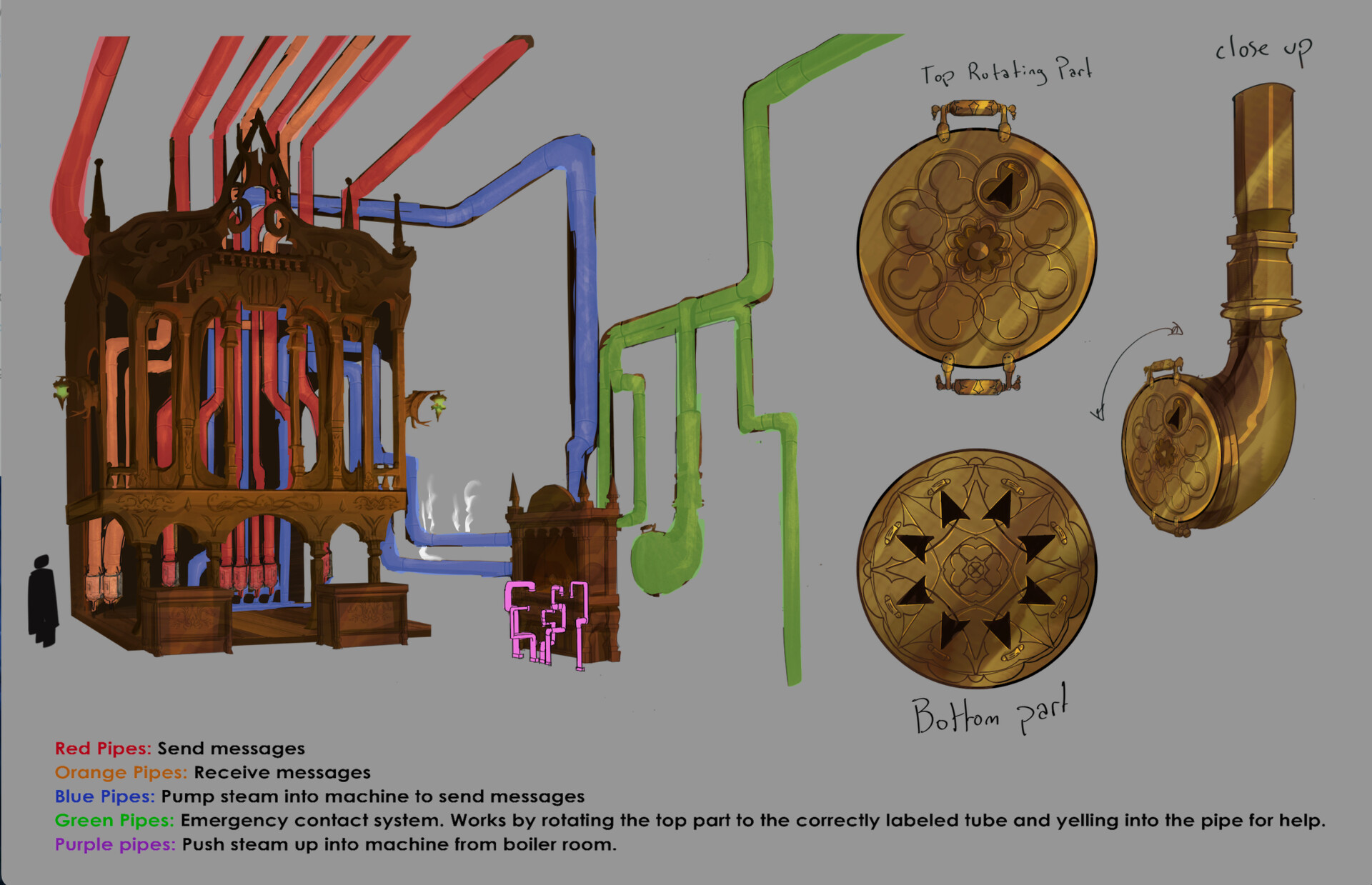The image is a detailed, hand-drawn schematic of an old messaging machine, possibly used in businesses to transport messages through an intricate network of color-coded pipes. The background is gray, and on the left side, an elaborate, full-color diagram of the machine is displayed. This machine features numerous pipes, each serving a specific function: red pipes send messages, orange pipes receive messages, blue pipes pump steam into the machine to send messages, green pipes are part of an emergency contact system activated by rotating the top part of the labeled tube and yelling into it, and purple pipes push steam up from the boiler room.

On the bottom left, a color-coding key outlines the function of each pipe. The right side of the image includes close-up cross-sections of various fixtures made of brass, labeled as "tap rotating part," "bottom part," and "close up," showing the intricate details of the pipe system. This schematic provides a comprehensive view of how messages were transported using pressurized air or steam, with a particular emphasis on the function and flow of each colored pipe throughout the machine.